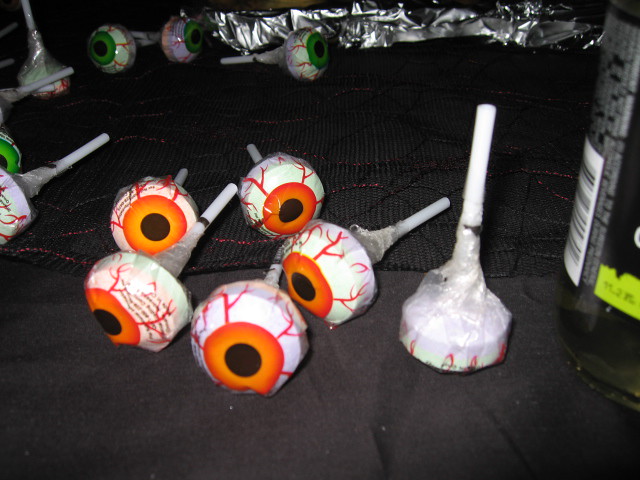The image depicts an assortment of Halloween-themed eyeball lollipops arranged on a black tablecloth adorned with red and black wavy lines. The lollipops feature a white candy base with cylindrical shapes, wrapped in plastic that mimics bloodshot veins with vibrant red lines. Each "eyeball" has a central black pupil surrounded by an iris, mostly orange but with several green variants visible in the background. A total of seven lollipops can be clearly seen, with one positioned upside down. The lollipops appear to be intended for trick-or-treaters, perhaps left out on a porch for convenience. To the right side of the arrangement, a partially visible bottle with a black body and light green labeling adds to the scene’s festive ambiance.